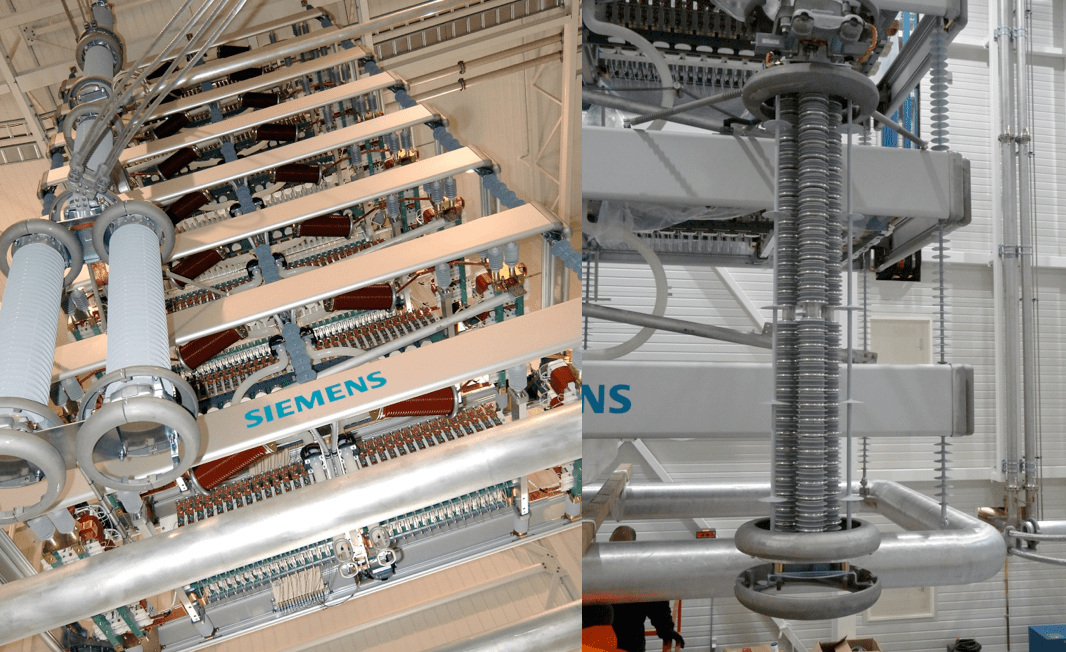The image is composed of two side-by-side photographs featuring complex electrical machinery manufactured by Siemens (S-I-E-M-E-N-S). The left photograph is in color with a slight orange tint, likely due to lighting, and showcases a sophisticated machine with a series of seven vertical metallic bars or rungs resembling a ladder. Spiraled cylinders or rolling mechanisms with gray circular ends are mounted on these bars, connected to a metal rigging that houses various electronic components, including circuit boards and insulators. The entire assembly is indicative of an advanced electrical installation. The right photograph, although appearing monochromatic at first glance, reveals color upon closer inspection, showing more detailed views of the same or similar machinery from a different angle. Here, the components are primarily silver or gray, with blue and red hints. A close-up of one of the coils is visible, displaying a silver metallic coiling within a casing with three large silver or gray circles encircling it, attached to a swing arm. The setting appears to be inside a white-walled factory, with additional elements such as boxes at the base and pipes running down the wall, and possibly a person visible at the bottom.